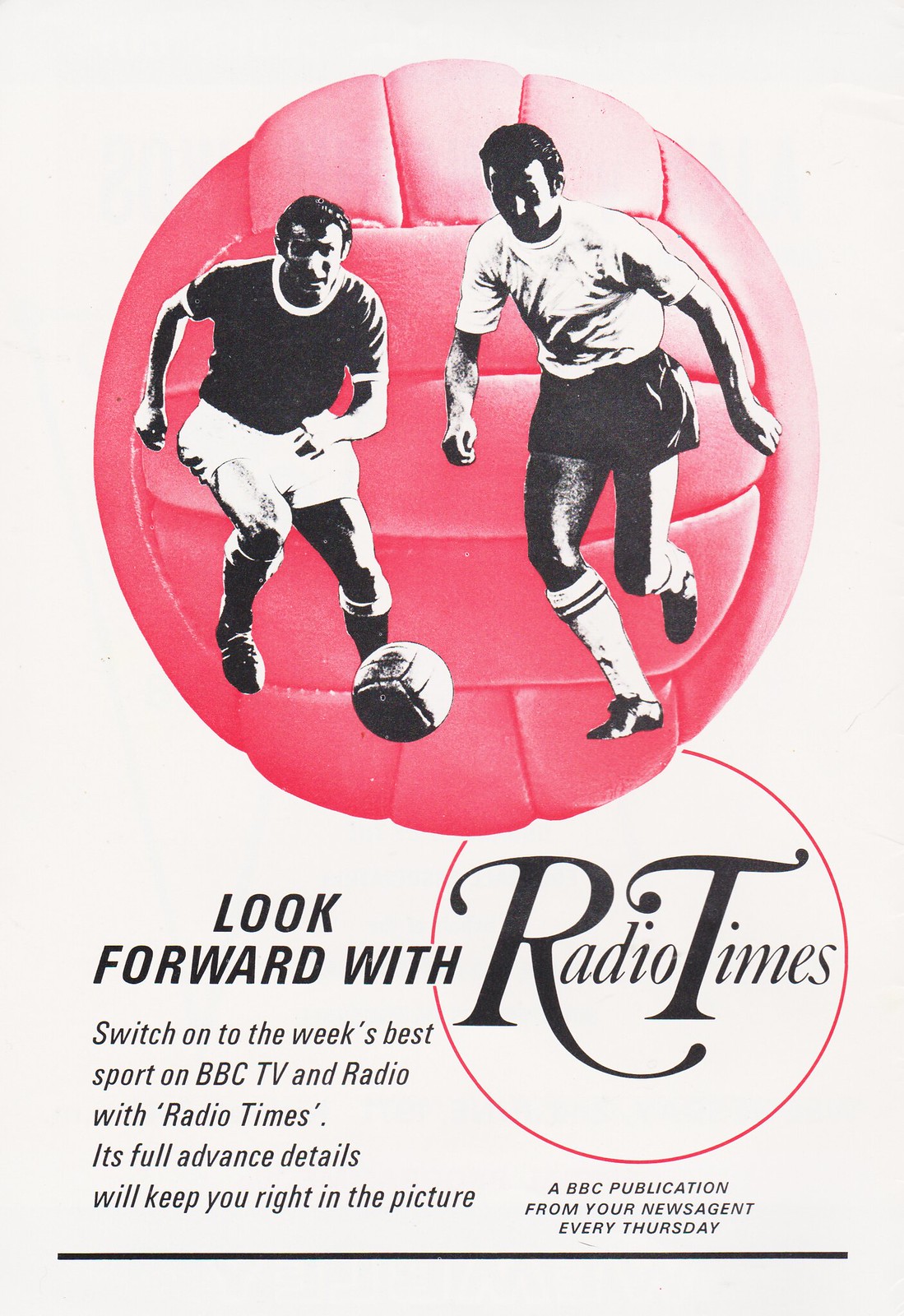The image is a detailed advertisement poster with a background that transitions between pale blue and pale pink hues. Dominating the top half of the poster is a prominent pink soccer ball. Superimposed on the soccer ball is a black and white image of two soccer players, mid-action, seemingly confronting each other in their attempt to kick the ball. Below this dynamic scene, the text reads in varying fonts and colors, "Look forward with Radio Times." The phrase "Radio Times" is encircled with a pink line. Beneath this, another line of text invites viewers to "Switch on to the week's best sport on BBC TV and radio with Radio Times. Its full advanced details will keep you right in the picture." Further down, it states, "A BBC publication from your news agent every Thursday," with a thin black line running horizontally across this section, emphasizing the information. The ad highlights both the thrilling action of soccer and the comprehensive sports coverage offered by Radio Times, a BBC publication.